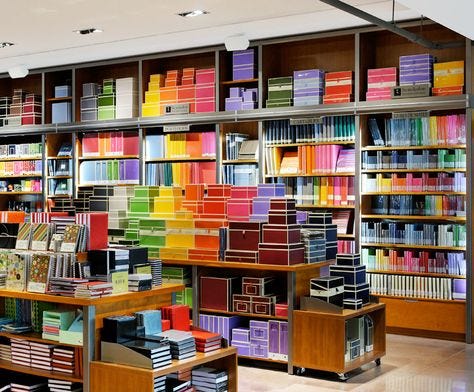This photograph captures the vibrant interior of a paint or hardware store specializing in painting and creative materials. Dominating the scene are shelves stocked with an impressive array of colorful paper and small books, potentially sketchbooks or notebooks. The focal point of the image is a large shelf extending to the ceiling at the back, meticulously arranged in a dazzling spectrum of colors including red, blue, green, violet, among others, reminiscent of a perfectly ordered rainbow. In front, two smaller shelves display an equally vivid assortment of products, giving the impression of a well-stocked and aesthetically pleasing craft or school supply section. The angle of the shot, taken from the right side, suggests the perspective of a customer or store employee keen to showcase the vibrant and orderly setup of the store’s offerings.